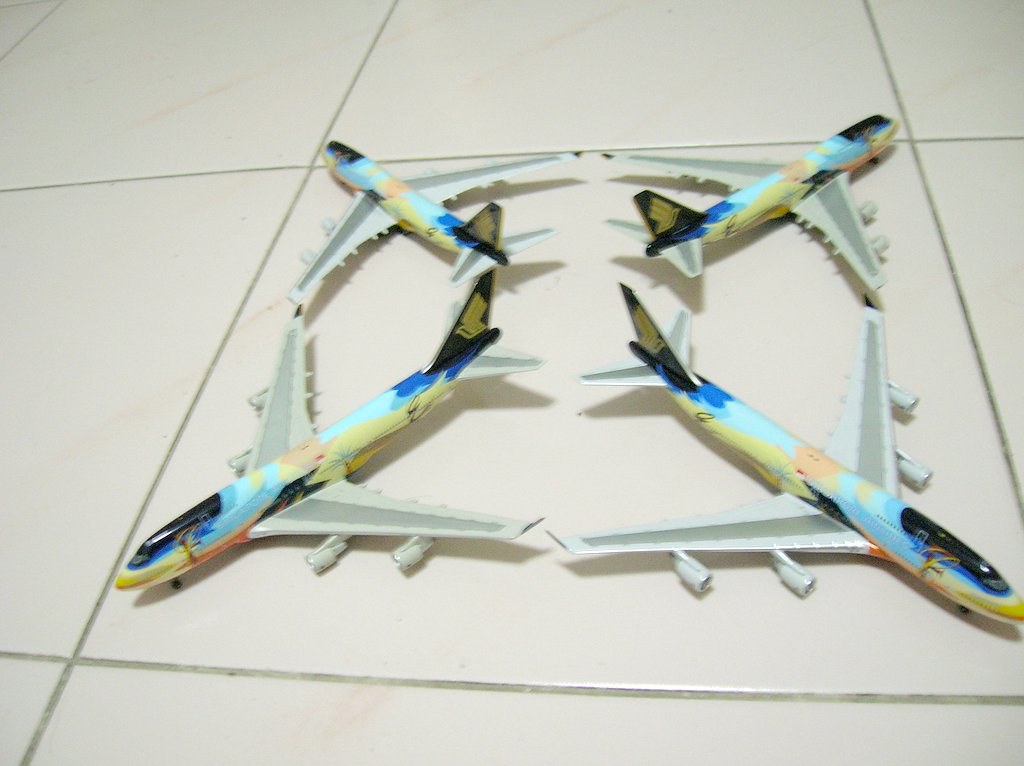This is a detailed horizontal photograph taken very close to a floor, capturing a section of what seems to be light beige ceramic tiles with darker gray grout. In the center tile, four small, realistic-looking model airplanes are positioned with their noses pointing towards the corners of the tile, nearly touching wings and tails. Each airplane features gray wings with a dark gray stripe along the center and a black cockpit and tail. The bodies are adorned with vibrant, irregular patches of light blue, dark blue, pale yellow, pink, and pale orange paint. Although there are gold emblems on their tails and possibly other text on their bodies, the details are not clear enough to distinguish. The artistic display of the planes contrasts against the plain, light-colored tile, creating a visually intriguing scene.